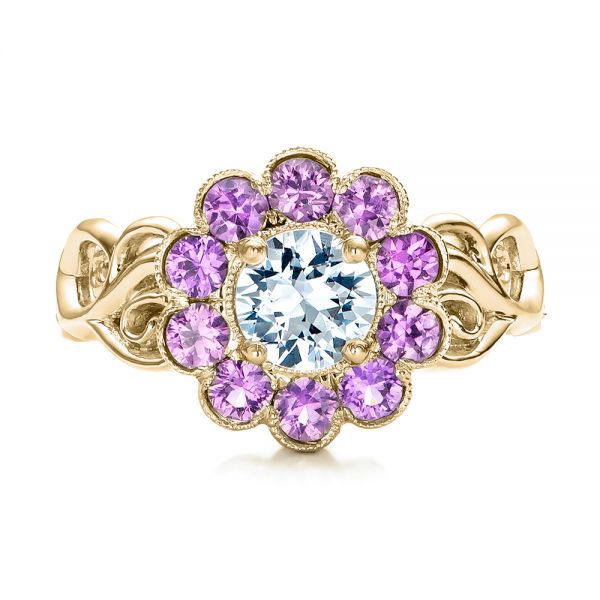This photograph showcases an ornate and exotic gold ring set against a solid white gradient background. At the heart of the ring lies a prominent, large diamond held in place by four gold prongs. Encircling this central diamond are ten lavender-colored gemstones, meticulously arranged to create the illusion of flower petals. This floral motif, with the central diamond as the flower's core, is enhanced by the petal-like formation of these gemstones. The ring itself features a flowing pattern of intermeshed and crisscrossing gold swirls, reminiscent of a vine wrapping around the finger. This intricate design not only accentuates the flower likeness but also adds to the ring's elaborate aesthetic. The high-shine gold metal forms the ring's base, providing a cohesive, luxurious setting that complements both the central and surrounding stones.